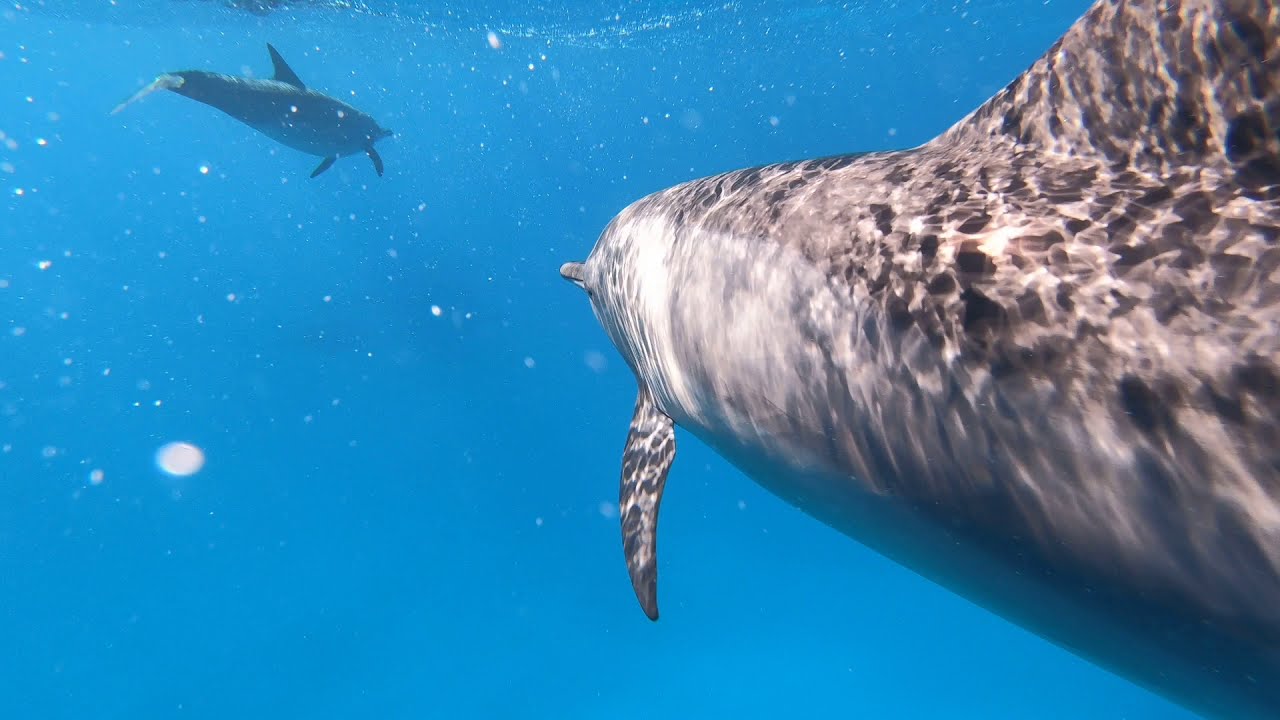The image captures an underwater scene featuring two dolphins swimming in the ocean. The photograph appears to be taken with a GoPro camera, potentially attached to the fin of the dolphin on the right, providing a close-up perspective from just behind it. The dolphin on the left is further ahead, shaded in dark blue, gracefully moving through the serene, light blue ocean waters speckled with white, which might be particles or light reflections. The sun's rays filter through the water, illuminating the dolphins and giving the scene a tranquil, almost ethereal quality. The photo is devoid of any other visible creatures or objects, focusing solely on the two dolphins as they swim close to the surface in the clear, middle-of-the-day sunlight.